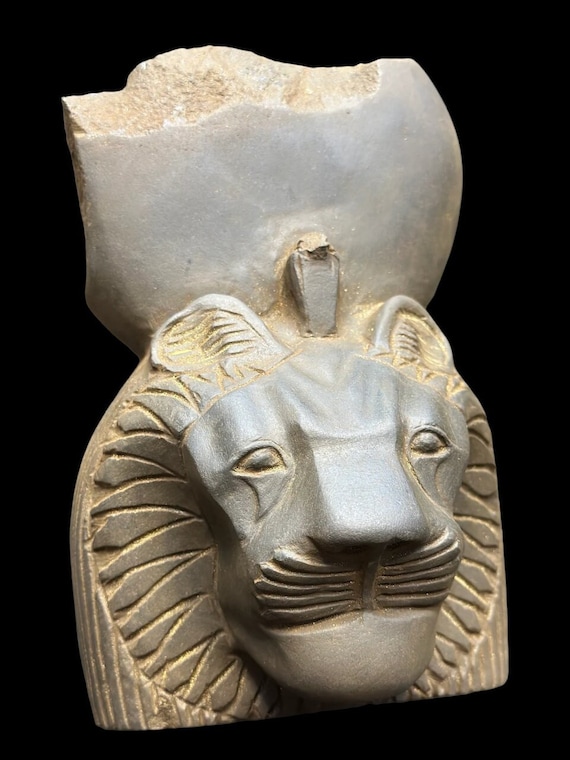This image displays a detailed stone statue set against a solid black background. The statue, standing at approximately a foot and a half tall, depicts the intricately carved face of a lion, complete with a mane, whiskers, eyes, and ears. The material of the statue appears to be a mix of light gray and tan, giving it a sandy texture. The lion's face is positioned at the bottom of the statue, while the top features a large, cracked circular boulder. The coloration transitions from a more orange hue at the bottom to a lighter color rock at the top, suggesting the statue's aged appearance. There are specific carved details, including five distinct lines on each side of the lion's nose, which enhance the lifelike representation of the creature.